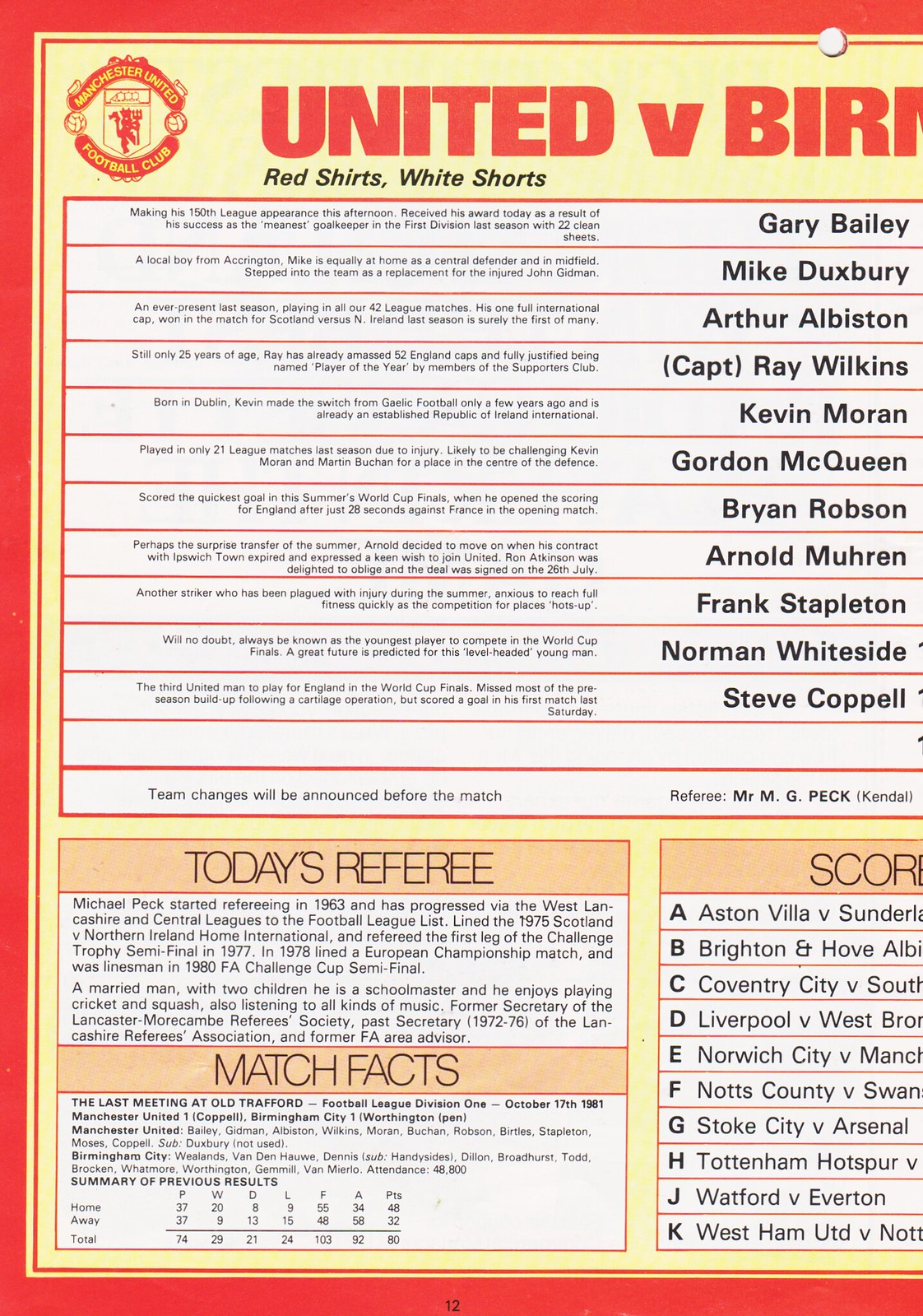The image is a vertically aligned, rectangular segment of a sporting program with a distinct red border. The top of the page prominently features the partially visible title "United v BIRM," which indicates a match between United and a team starting with "BIRM." Below the title, there is a description stating "red shirts, white shorts," likely denoting the uniform colors of one of the teams. 

The page is structured with multiple text columns. On the left-hand side, there is a narrow column of small, right-aligned text, presumably detailing information about the teams or event. Adjacent to this column is a list of player names in larger, black print, each separated by a red line. This list starts with Gary Bailey and ends with Steve Koppel.

At the bottom of the image, there are two sections in all caps black text. The first is titled "TODAY'S REFEREE," which includes a couple of paragraphs likely containing a bio or details about the referee. The second section is titled "MATCH FACTS" with additional left-aligned information under it. To the far right, there is a partially cut-off table labeled "SCORE." This table lists teams alphabetically from A to K with their respective matchups, including "Aston Villa vs. Sunderland" for 'A' and "Brighton" for 'B', indicating previous match scores or fixtures.

The background color of the page is yellow, and there is an orange border around some elements, including a logo to the left of the "United v BIRM" title. The structured layout and color highlights indicate it's an informative and organized sporting program.